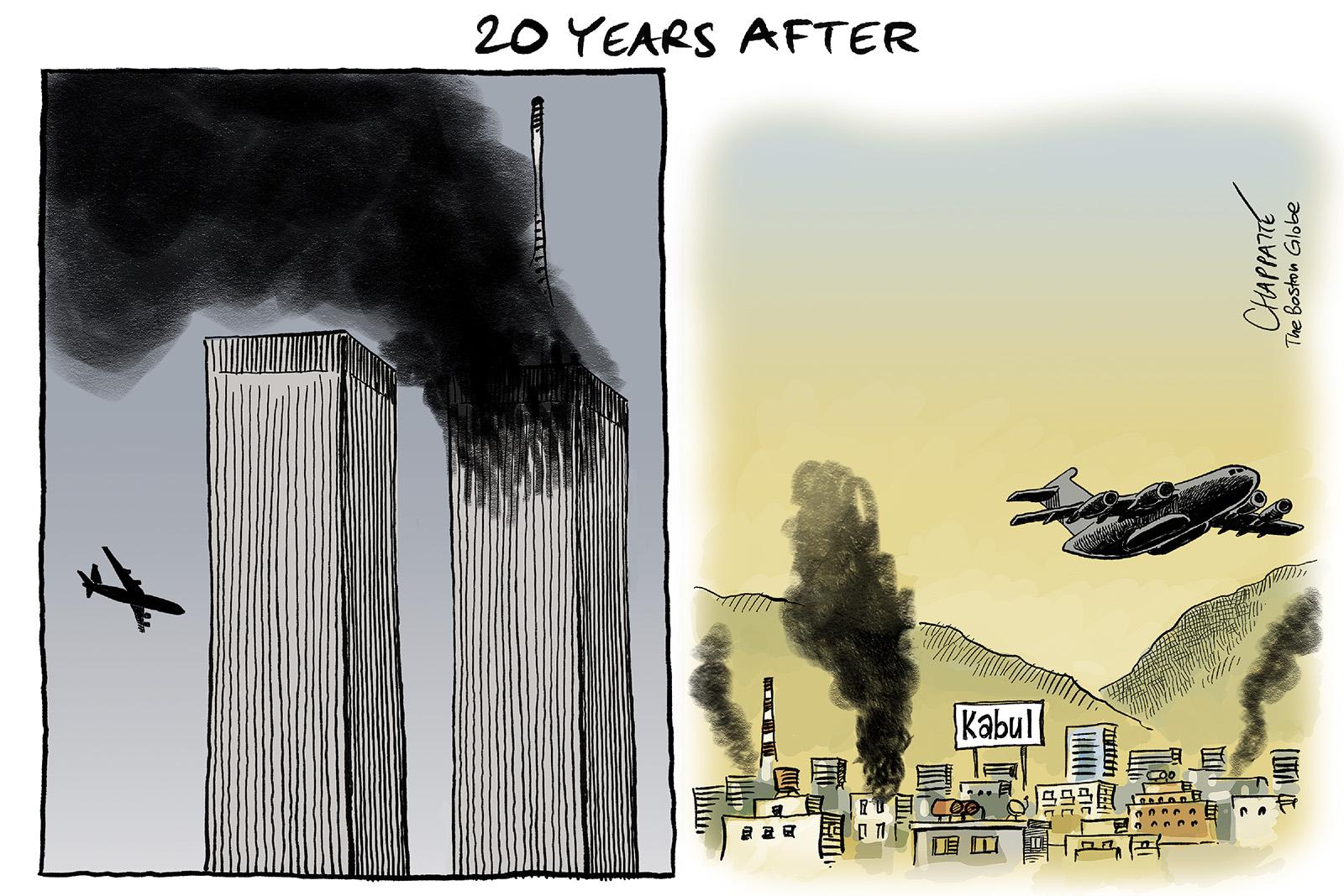The image is a political cartoon with a dark-colored backdrop divided into two panels, each marked by the headline "20 years after." The left panel is an evocative sketch depicting the fateful moment of the September 11th attacks on the World Trade Center. It illustrates the iconic twin towers, with intense black smoke billowing from the right tower as a dark plane is seen approaching the left tower. The setting exhibits a haunting gray background, emphasizing the somberness of the event.

On the right panel, the scene shifts to Kabul, highlighted by a white sign with black lettering reading "Kabul" positioned above a cluster of buildings emitting dark smoke. Behind these structures, a vast airplane ascends into the bright yellow sky, with green hills or mountains visible in the distance. Further up in this panel, the artist's signature "CHAPPATTE" is noted sideways, accompanied by "The Boston Globe," identifying the creator's contribution to this piece. The juxtaposition of the two scenes poignantly reflects on the enduring impact of catastrophic events involving planes and smoke, separated by two decades.